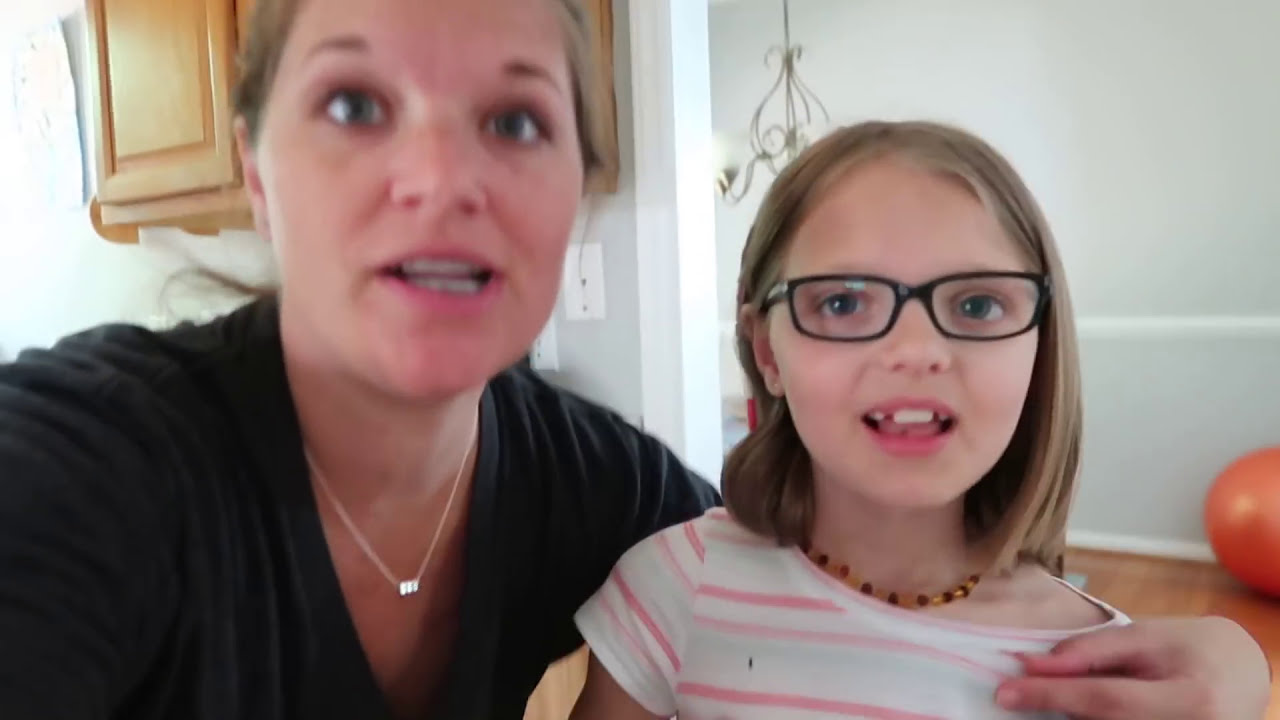In the image, a fair-skinned adult woman and a young girl, both with blonde hair, are side by side, facing the front. They appear to be indoors, possibly taking a selfie or recording a video. The woman, on the left, has her left arm around the girl’s shoulder and is wearing a dark long-sleeved shirt along with a delicate silver necklace featuring a shiny rectangle pendant. Her mouth is slightly open, as if she's about to speak. The girl, on the right, is in focus, wearing black-framed glasses and a pink and white striped shirt. She has a cheerful expression, showing her top two recently lost teeth. The girl is also adorned with a brown and tan necklace. In the background, there's a light tan cabinet, some lights, and a chandelier hanging from the ceiling, contributing to the cozy indoor setting.